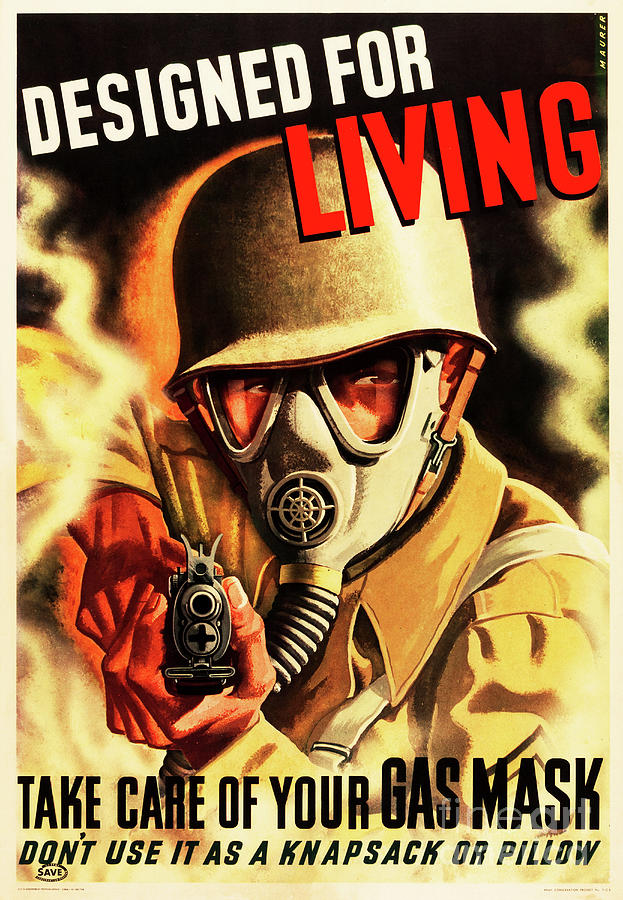The image is a detailed illustration of a WWII-era poster featuring a soldier equipped with a gas mask and pointing a gun directly at the viewer. The soldier, who has a beige helmet and a gray gas mask with two eye holes and a cylindrical respirator, appears serious and menacing. He is dressed in a brown WWII-era jacket with visible folds and a partially seen satchel indicated by a beige shoulder strap. The gun, held firmly with both hands, is black and gray, showing the muzzle and a bayonet attachment point. White wisps of smoke billow from both the left and right sides of the image, creating a dramatic atmosphere.

At the top of the poster, in slanted white text, are the words "DESIGNED FOR," while just above the helmet, in bold red text, it reads "LIVING." The majority of the poster's space is dominated by the depiction of the soldier. At the bottom, the text in black, bold font states: "TAKE CARE OF YOUR GAS MASK. DON'T USE IT AS A KNAPSACK OR PILLOW," with the word "SAVE" in the bottom left corner. The overall warm color palette ties the elements together, emphasizing the gravity of the warning for soldiers to properly maintain their gas masks.